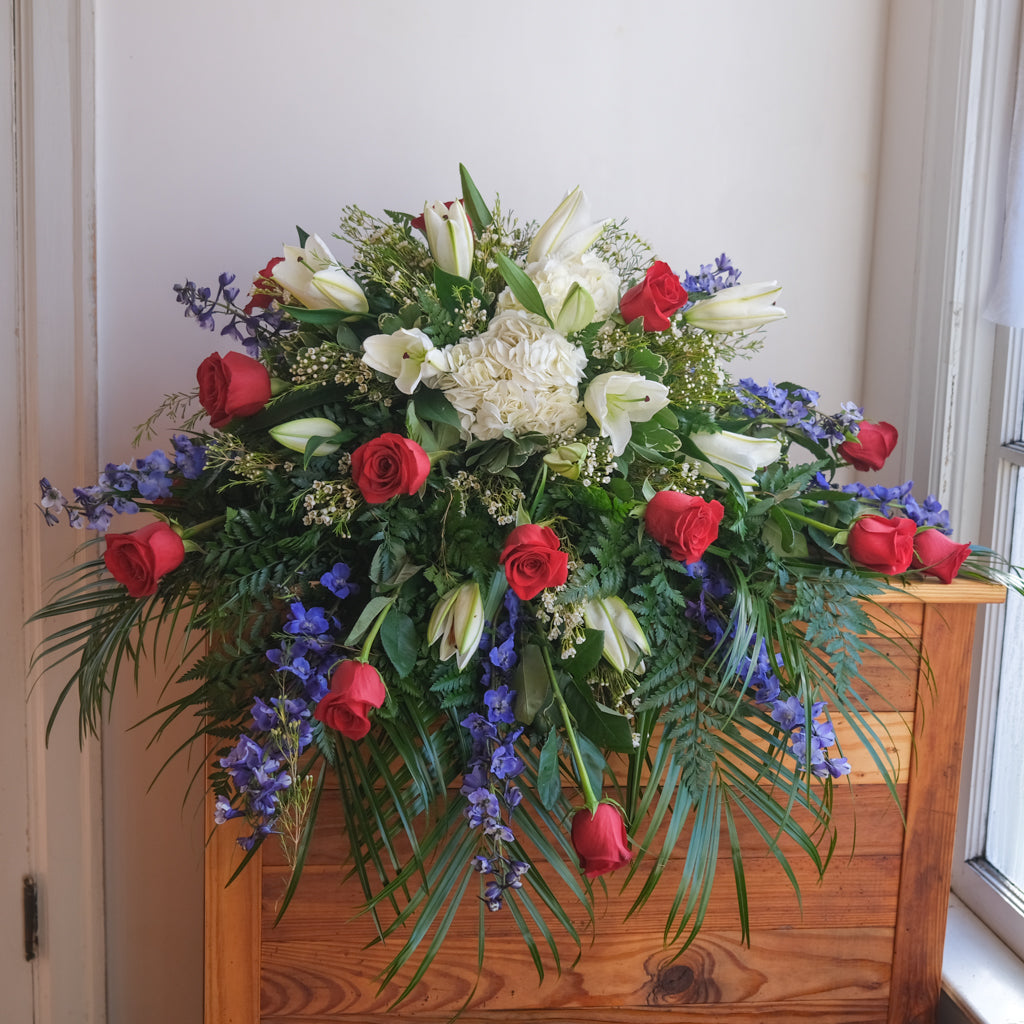In this realistic photograph, we see a brightly lit, white room featuring a medium-stained wooden dresser positioned beneath an open window. The dresser is adorned with a large, elaborate floral arrangement that resembles a casket spray or a substantial wedding centerpiece. This bouquet includes a vibrant mix of red roses, white tulips, blue flowers, and clusters of white carnations, alongside abundant greenery and some yet-to-bloom buds. The detailed setting reveals door hinges to the right, a window with a curtain or blind on the left, and natural sunlight pouring in, illuminating the room's stark white walls and highlighting the striking display of mixed blooms.